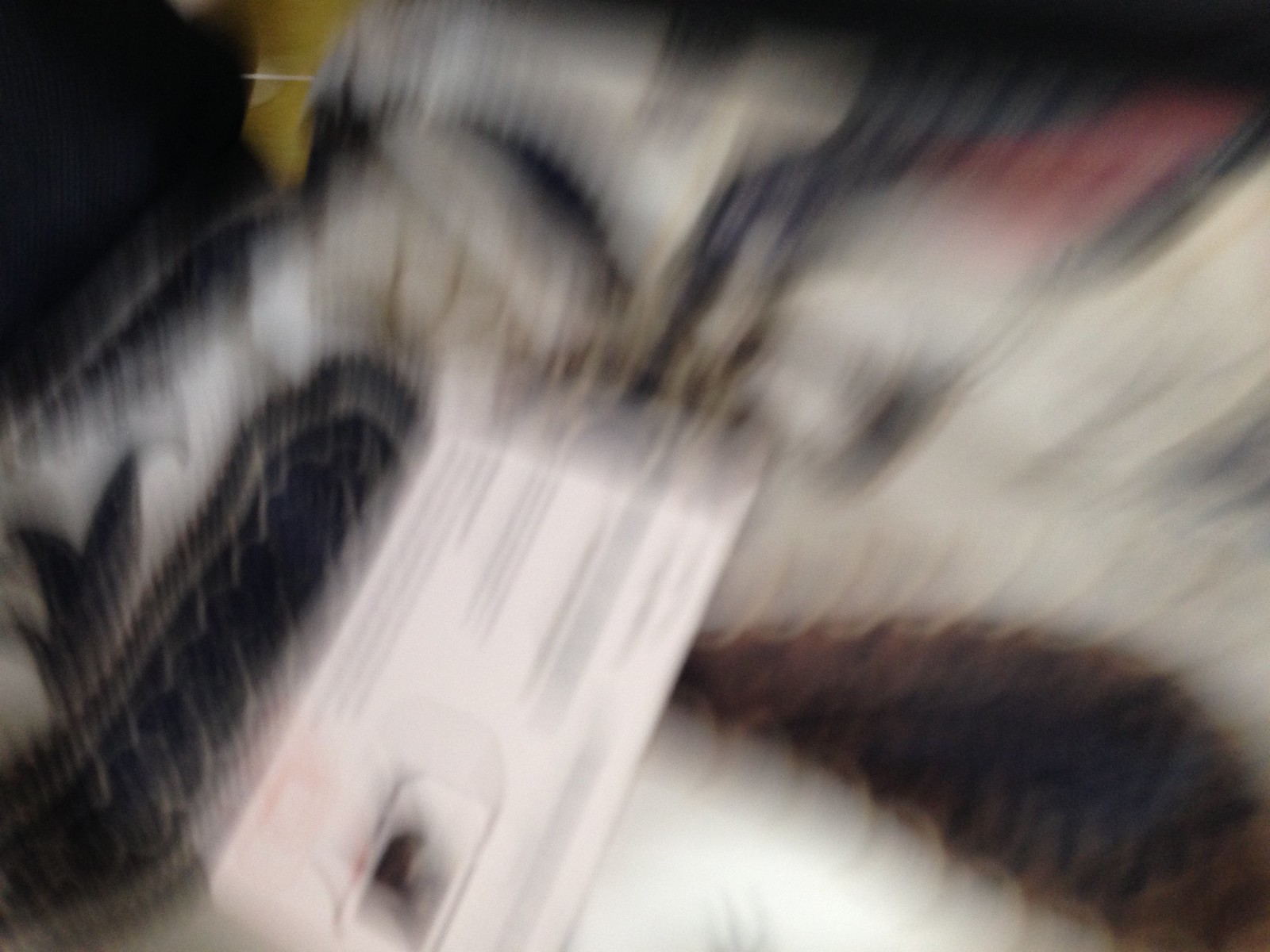This image appears to be a blurred photograph depicting an indoor scene. Central to the image is what seems to be a door, slightly off-center. Surrounding the door is a variety of fabric textures and patterns, which suggest a cozy, lived-in environment. In the foreground, it looks like the photograph was accidentally taken, likely by someone sitting on a couch with a blanket draped over them. The perspective suggests the person was holding a cell phone in their lap when the image was captured. The device seems to be an Android phone, possibly a Samsung or Nokia, as indicated by the central placement of the camera. The overall impression is informal and candid, perhaps taken during a moment of relaxation or while playing a card game.